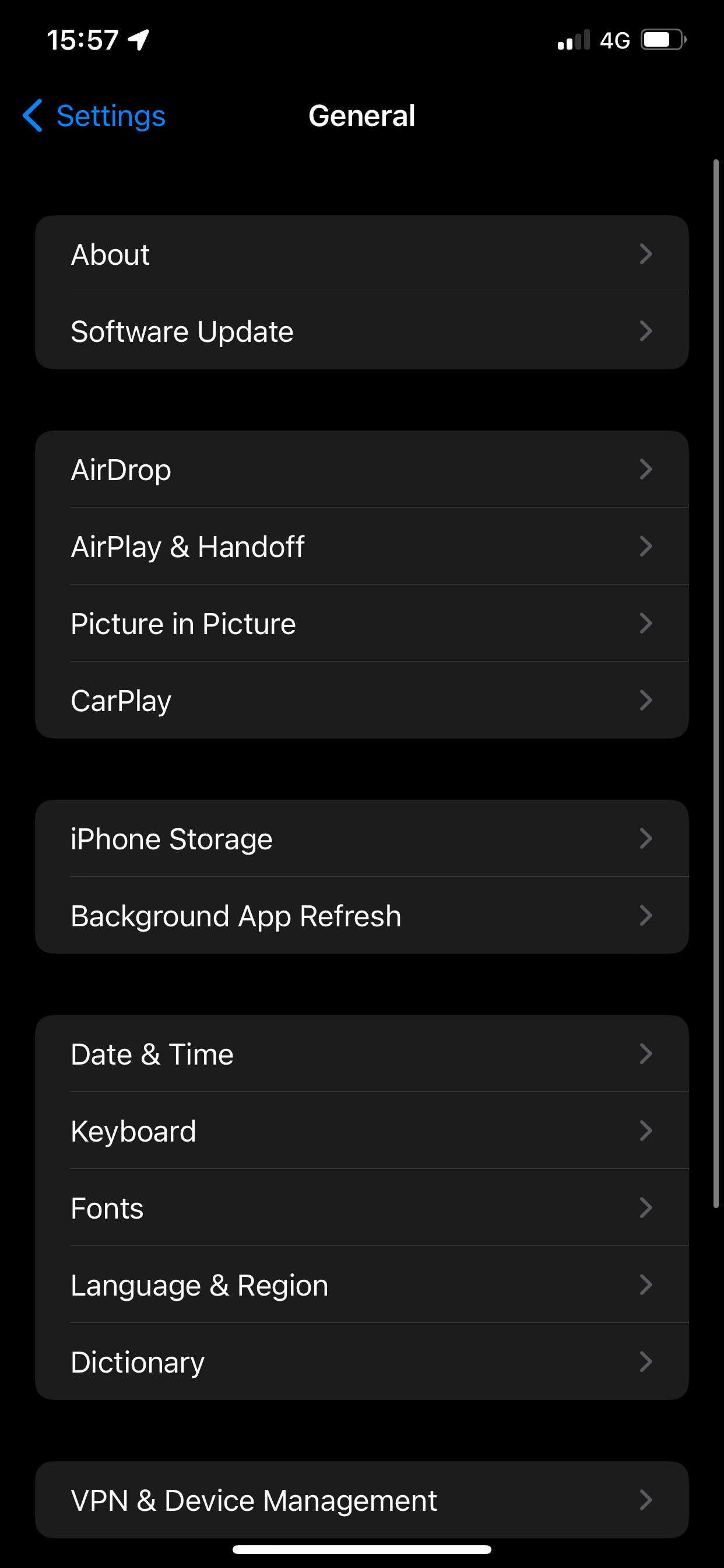This vertically oriented screenshot captures the "General" settings menu on a smartphone, showcasing various system options. On the top left, the time is displayed as "15:57" in military format, accompanied by a white arrow. The top right corner indicates a "4G" network connection, along with icons for battery status and Wi-Fi signal. Centered at the top, the word "General" is presented in white text, while "Settings" in blue text with a left-facing arrow appears on the left side.

Beneath this header, the screen contains a series of darker gray boxes, each representing a different settings category. The categories are listed vertically along the left side and include:

- About
- Software Update
- AirDrop
- AirPlay & Handoff
- Picture in Picture
- CarPlay
- iPhone Storage
- Background App Refresh
- Date & Time
- Keyboard
- Fonts
- Language & Region
- Dictionary

Each category name is followed by a small gray arrow pointing to the right, indicating additional nested options.

Towards the bottom, there is another tab labeled "VPN & Device Management," also with a right-facing arrow. A thin gray vertical line occupies a portion of the right side border, and a thicker white horizontal line is positioned at the bottom center of the screenshot. The overall design and layout are typical of a mobile device's settings interface, providing a comprehensive overview of general system settings.